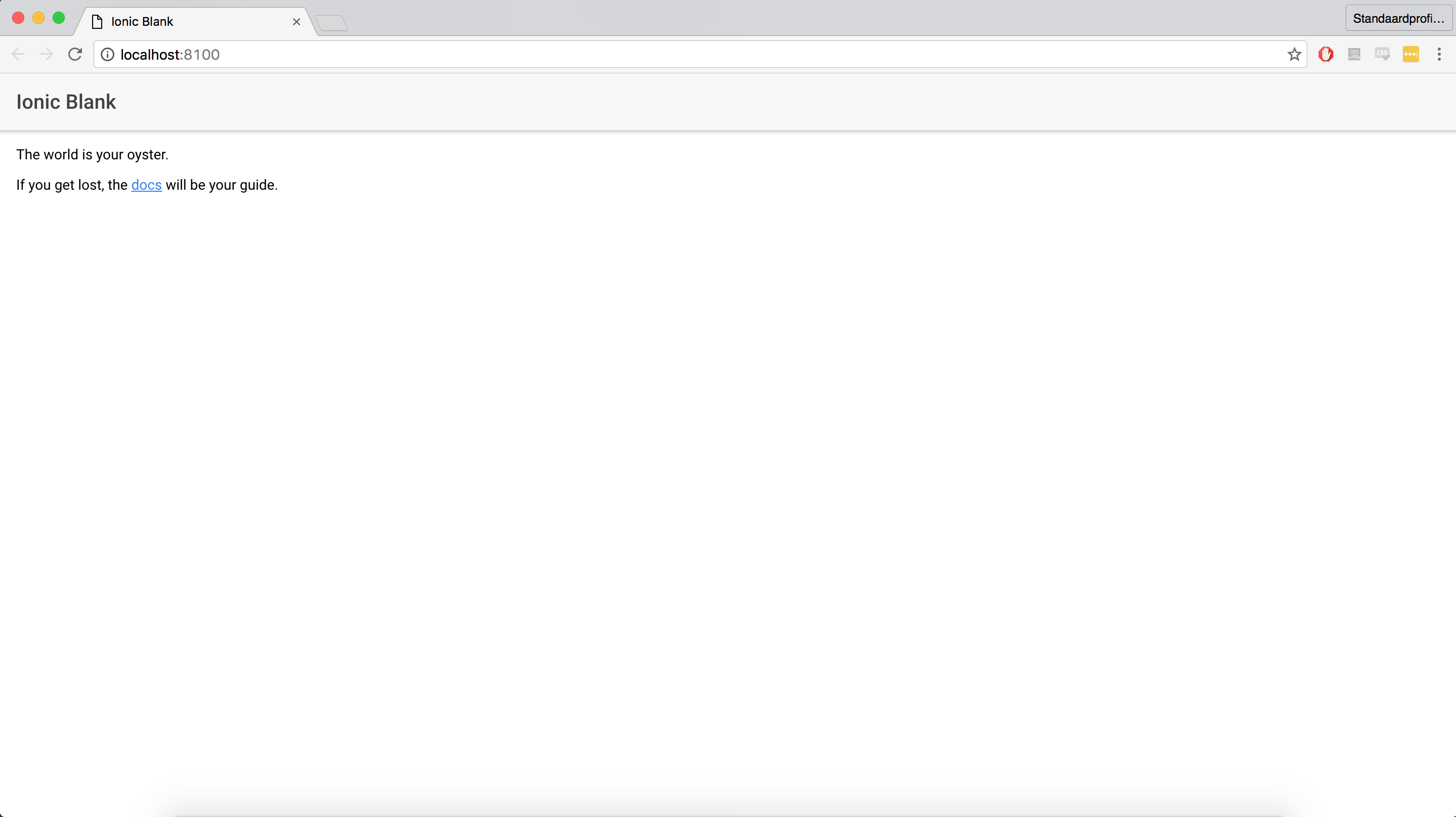This seems to be a visual description of a browser window on an Apple iMac, likely showing a development or local testing environment for an Ionic application. Here’s a cleaned-up and detailed caption:

---

The image depicts a browser window, distinguished by a dark grey bezel typically associated with Apple iMac interfaces. On the top left of this bezel, three circular buttons are visible: one red, one orange, and one green, indicating the classic Mac controls for closing, minimizing, and maximizing the window. On the top right of the bezel, the standard profile icon is partially visible alongside an ellipsis icon, suggesting additional options.

Within the browser window, a single tab is open, displaying a document icon next to the text "Ionic blank" in black. To the right of this tab label is a black 'X' for closing the tab, followed by grey left and right arrow icons for navigation, a refresh symbol, and a URL bar. The URL bar contains an icon of a black circle with a white 'i' in its center, alongside the bold text "localhost" followed by ":8100" in a white field. Also within the URL bar are a black star icon, a red circle with a white gloved hand icon, a dark grey square, a mid-grey square with a dark grey border, and an orange square containing three white ellipses, signifying various functionalities. 

On the left-hand side of the window, a mid-grey section features the bold black text "Ionic blank." Below it, within a blank white space, the phrase "The world is your oyster" is written in black text. Following this is a new line: "If you get lost, the docs," with "docs" appearing in italicized blue, underlined to indicate it is a clickable link. The clickable "docs" suggests it provides guidance or further information.

---

Note: This description assumes the purpose is to convey a clear, comprehensive overview of the visual elements and layout of the browser window for those who might be visually impaired or unable to view the image.